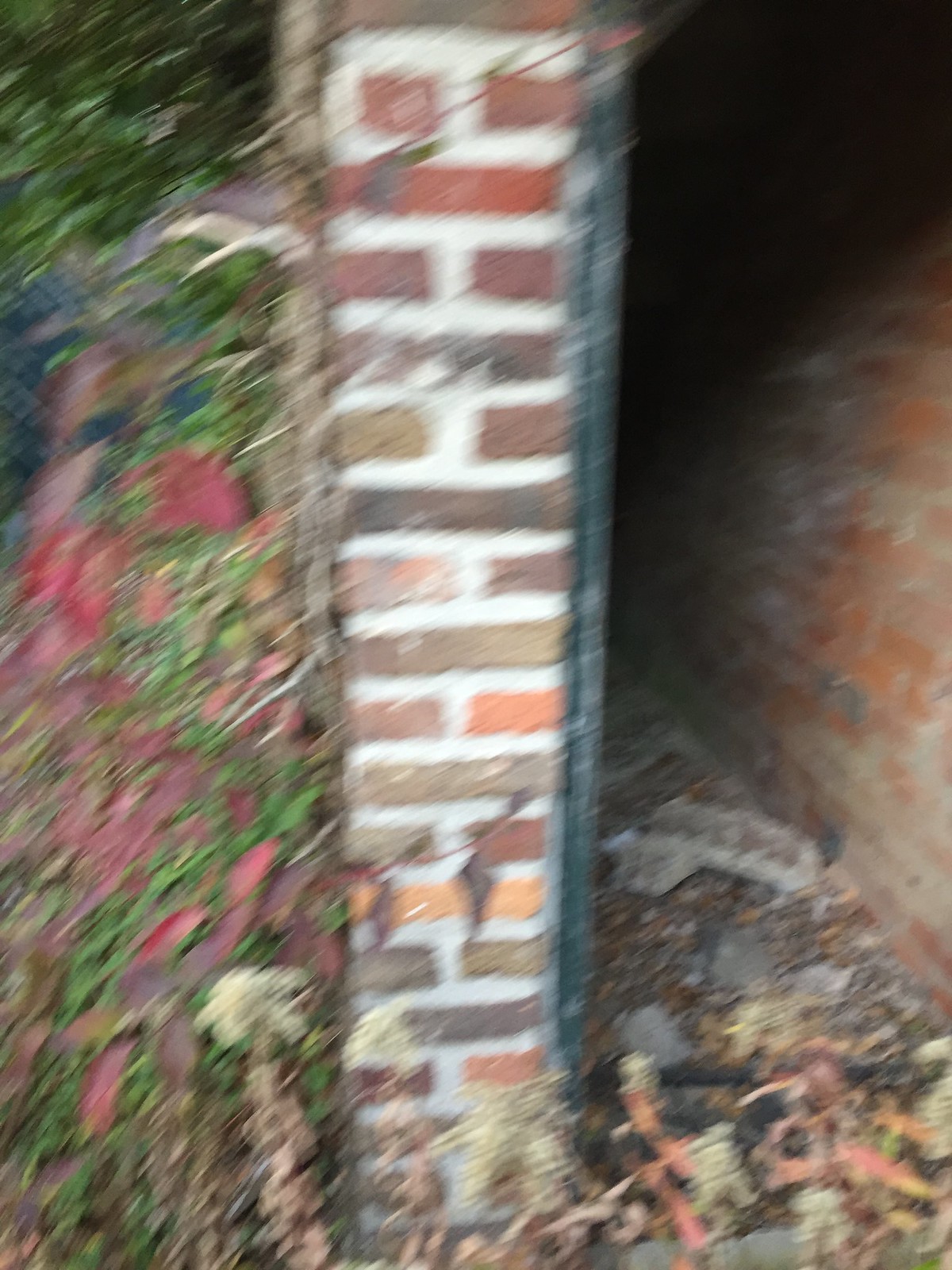The image depicts a very blurry side view of a dilapidated brick wall, with another parallel brick wall creating a narrow, almost room-like passage in between. Over time, the area has become heavily worn and neglected, featuring eroded bricks with significant amounts of concrete between them, some of which has fallen off. The ground in this enclosed space is littered with debris, including dirt, gravel, rubble, leaves, and small stones. To the left, there is some vegetation, possibly a rose bush or moss, growing up the wall, lending a sense of overgrowth and abandonment. The right side shows a black sheet or wooden attachment, which is hard to distinguish. Given its neglected state, the area is small but could be used to store items, although it now appears uninhabitable. Green trees are visible in the background, and the entire scene is enclosed by the two deteriorating walls.